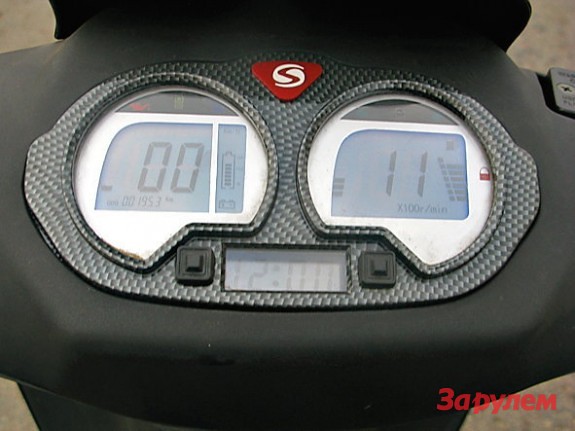This color photograph captures an intricate electronic device prominently positioned at the bottom right corner against a light brownish background. The device features a central area displaying the text "3APY" followed by script in a language other than English and the letters "EM". The upper midsection boasts an "S"-shaped logo. Adjacent to this logo are two circular screens: the left screen displays "00" alongside a nearly full battery icon, while the right screen reads "11". Below these screens are two black square buttons. Centrally located on the device is a middle screen displaying the time, "12:00". The device's exterior is predominantly black with a contrasting mottled grayish-silver outline resembling a pair of goggles. Additional detailing is provided by a black plastic-like material that outlines the top segment of the gadget.